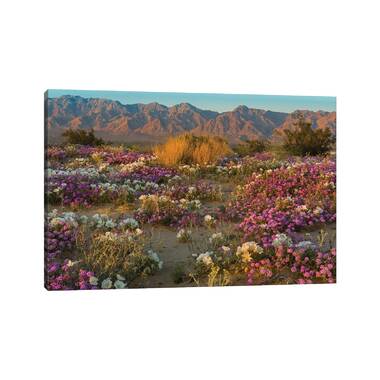The stunning outdoor image captures a vibrant desert landscape under a clear, blue sky, free of clouds. Dominating the background is a jagged, tan-gray mountain range with rugged, rocky faces devoid of trees but scattered with low brush. In the mid-ground, a lush valley extends, dotted with various cacti and blooming wildflowers in hues of purple, white, pink, and yellow, indicative of recent rains. Small trees with needle-like branches punctuate the scenery, adding texture to the otherwise arid environment. The foreground showcases a mix of dry grasses and colorful wildflowers, forming a picturesque tapestry that exemplifies the unexpected beauty of a well-watered desert. This scene is reminiscent of the Superstition Mountains near Florence, Arizona, a place steeped in legend and natural allure.